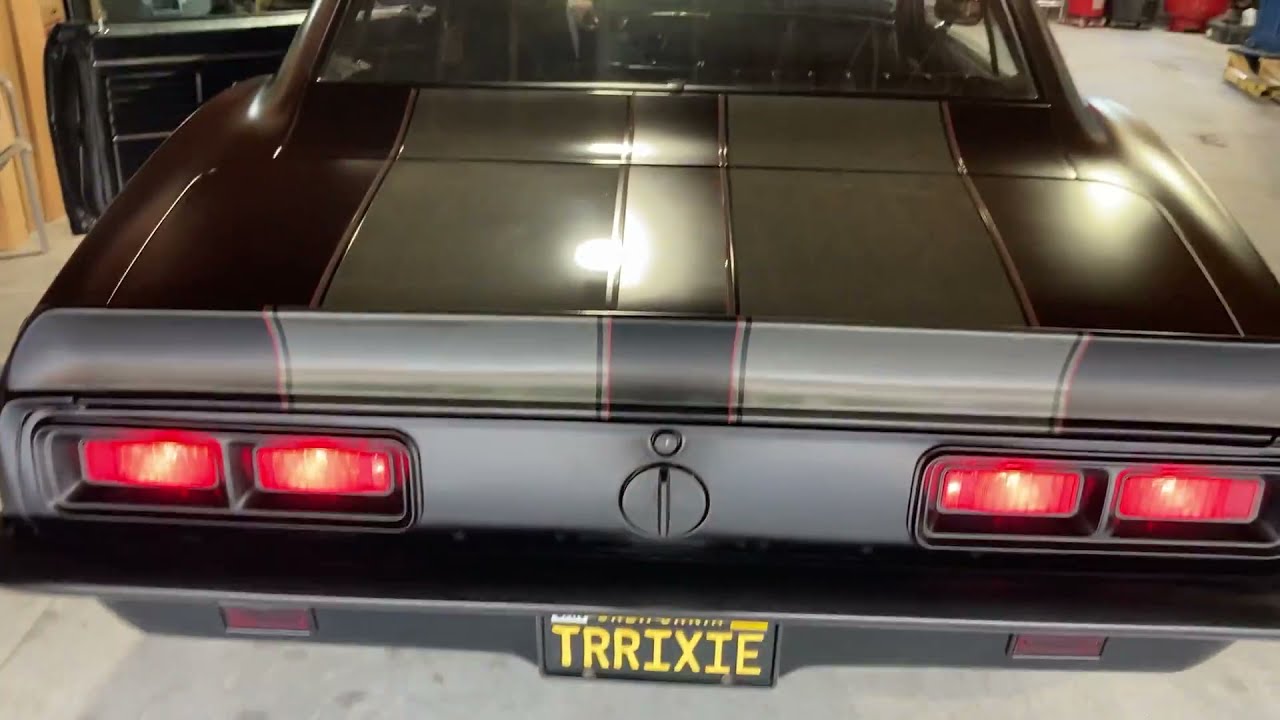The image showcases the rear view of a vintage-styled sports car, meticulously detailed with gray paint adorned with black stripes, accentuated by very thin red borders. This horizontally aligned rectangular photograph captures the car parked on a cement surface, likely inside a garage. The car's taillights are illuminated, displaying two bright red lights on each side. Prominently displayed in yellow letters on the visible license plate is the name "TRRIXIE." The driver's side door is ajar, but only the back window and part of the interior can be seen, hinting at a design akin to cars from the 70s. In the upper right corner of the image, concrete ground littered with unidentified items can be glimpsed, while the upper left corner hints at a wooden wall or door. The detailed texture and color scheme of the car, combined with the distinct vintage feel of the design elements like the lock mechanism, make it a striking homage to classic automotive aesthetics.